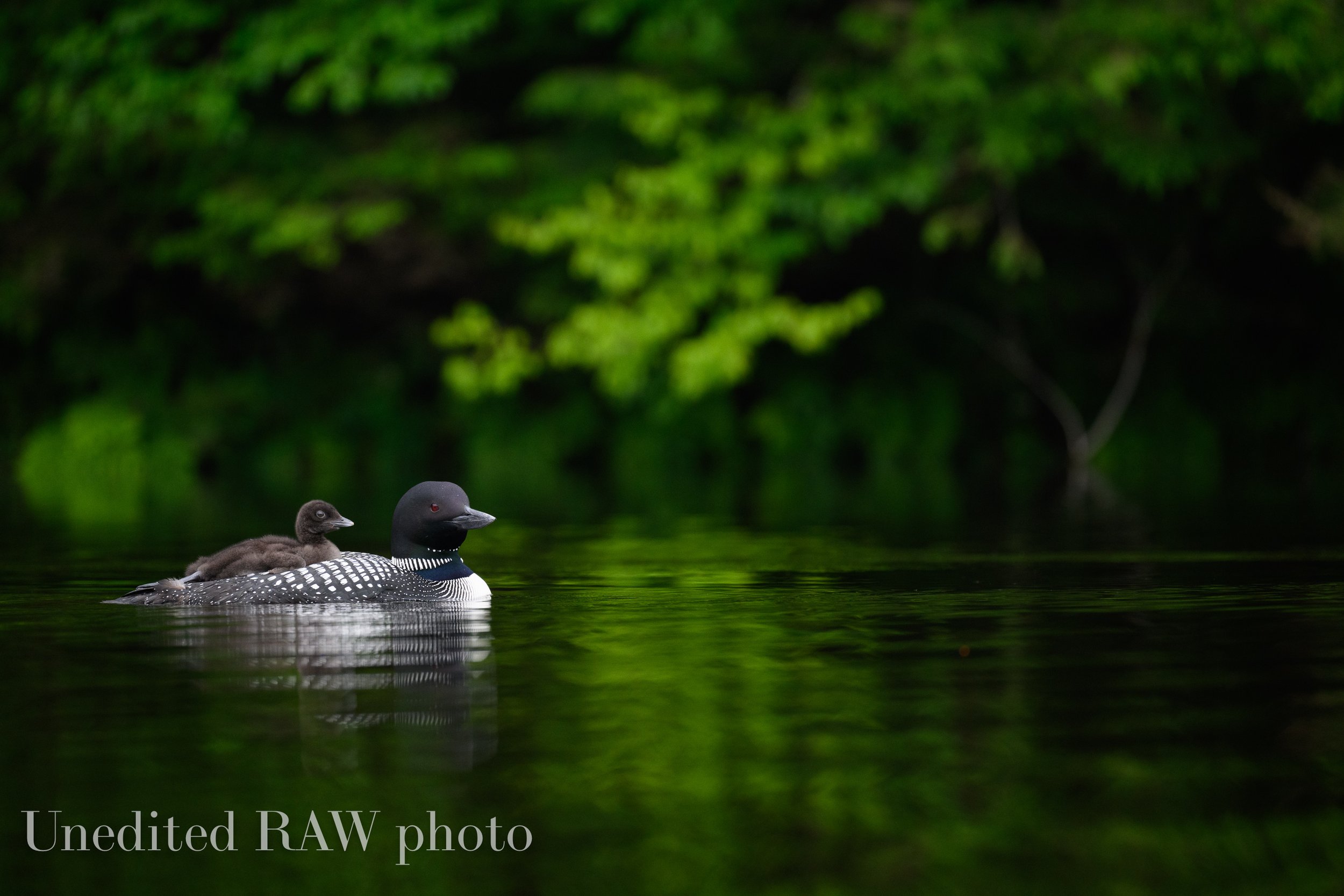The image is a horizontally aligned rectangular picture featuring an adult loon and its chick on a body of water. Predominantly, the upper portion of the image is filled with green leaves from a tree, while the middle and lower portions display water with gentle ripples. The water mainly appears black with hints of green reflections from the foliage above. Positioned on the left side, the adult loon, closest to the viewer, has a striking black head, a grey beak, and a brown beady eye. Its body showcases a black and white checkered pattern with white spots on the wings and a navy blue piece extending down to the chest, transitioning into more white and black stripes. Beside it, the chick is mostly dark brown and fuzzy, with black eyes and a light black beak, indicating it has not yet developed feathers. In the lower left corner of the image, light grey letters spell out "Unedited Raw Photo," with "RAW" capitalized.